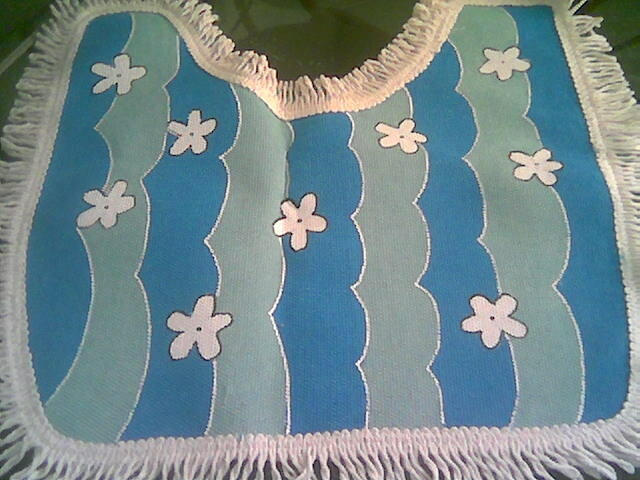The image is a detailed photograph of a fringed textile piece resembling a colorful bib. This fabric item lies on a green surface and features a distinctive design comprising light blue and light green wavy stripes, giving it a watery appearance. Dotted across these stripes are uniformly spaced white flowers, each outlined in black and featuring a central black dot. The shape of the textile has straight sides and a straight bottom with a U-shaped curve at the top, consistent with a bib-like outline. Encircling the entire piece is a white fringe, enhancing its decorative, homemade aesthetic. The white fringe and the meticulous detailing of the stripes and flowers suggest a crafted and possibly artistic quality to the fabric.